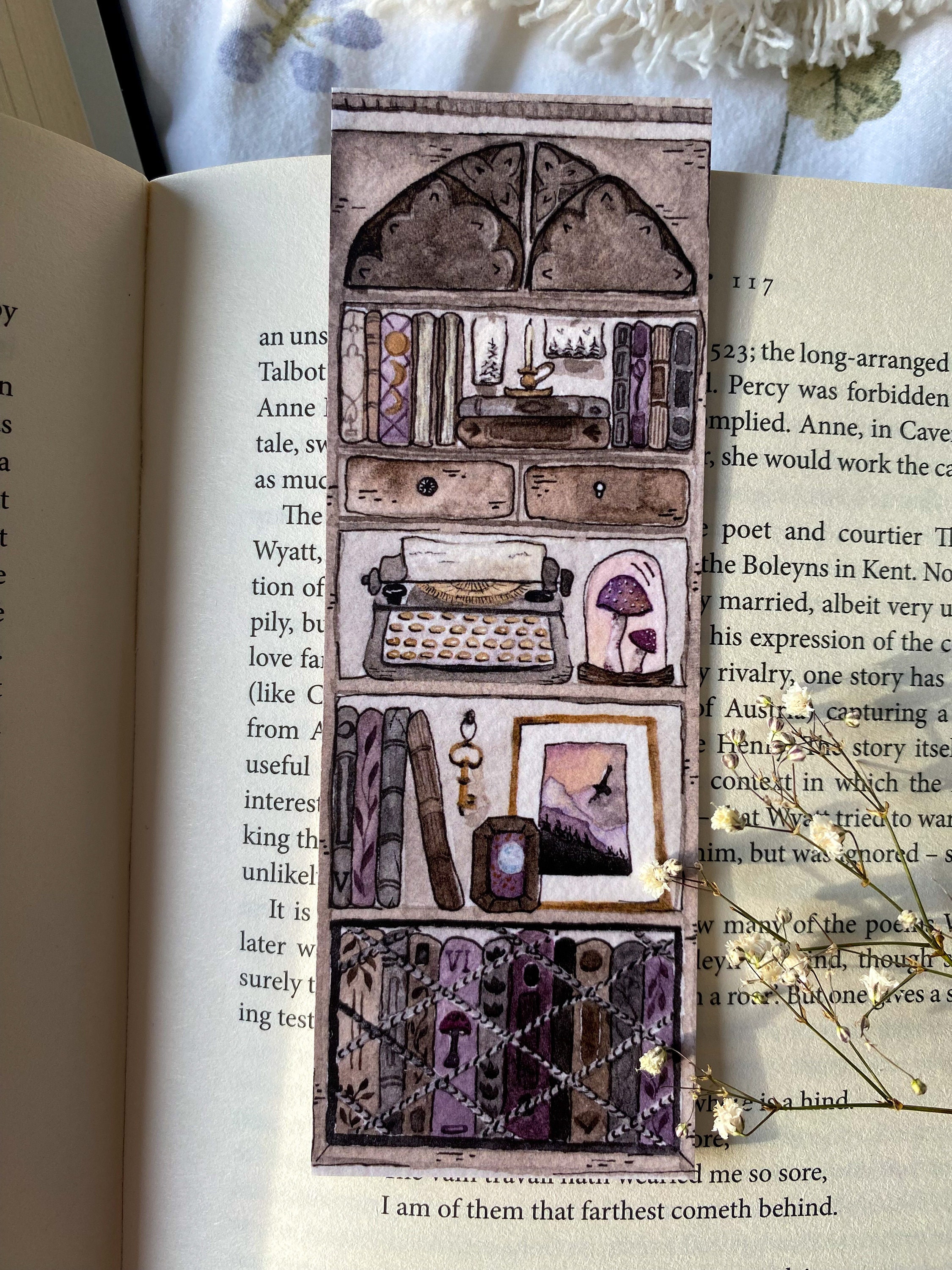The vertical photograph showcases an open book, primarily focusing on the right page. The white pages with black text contrast against a blue cloth background with dark specks. Dominating the central view is a beautifully detailed bookmark, reddish-brown in hue, dividing the page. It illustrates a whimsical bookshelf in five tiers, each adorned with intricate drawings. The top tier features a triangular-shaped window and clouds, followed by a bookshelf and desk with drawers and books, including a candle. The next section displays a typewriter beside a glass-covered mushroom, while below it shows a key on a hook, a framed picture of a bird over a mountainous scene, and more books. The final tier reveals multiple book spines hidden behind a crisscross, cage-like pattern. Complementing this serene bookmark scene is a delicate branch with tiny white flowers, likely baby's breath, intruding from the right side. The image suggests a cozy, reflective atmosphere, with the hand-drawn bookmark as the focal point amidst the open book's simple, off-white pages.